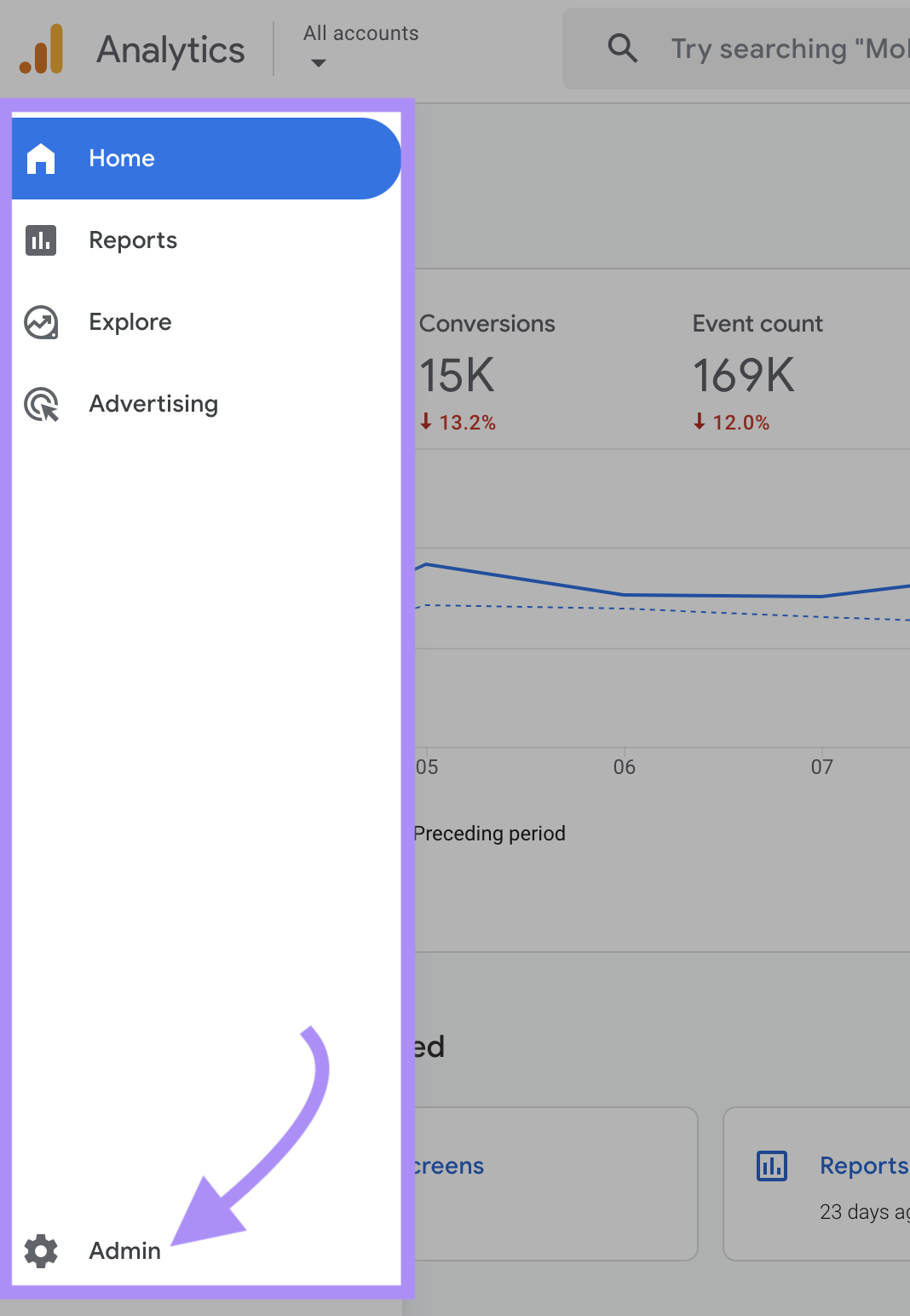This detailed color image showcases various elements of a web analytics dashboard. At the forefront is a white pop-up box or control box edged with purple, featuring a hand-drawn purple arrow, suggesting user interaction, possibly for page selection or navigation. This pop-up partially obscures the grayed-out web page behind it.

The main dashboard is dominated by a section labeled "Analytics" at the top, presenting three vertical columns in varying sizes—small, medium, and large—in gradients of red and orange. These columns potentially represent different datasets or metrics. Adjacent to this, at the top of the page, are options to view "All Accounts," and there is a "Search Box" with the prompt "Try Searching."

Prominent statistics are displayed: "Conversions" at 15K, indicating a decrease of 13.2%, and "Event Counts" at 169K, down 12.0%. Beneath these statistics, partially obscured by the pop-up box, is a graph featuring two blue lines, which likely shows trends over a "Proceeding Period."

On the left side of the screen, the pop-up box covers almost half of the webpage. A hand-drawn, curving arrow points towards the "Gearbox" and "Admin" settings, suggesting areas for further configurations or settings adjustments. In the top left corner, the navigation includes a blue rectangle highlighting "Home," with "Reports," "Explore," and "Advertising" options listed below in black text against a white background.

The overall layout and elements indicate that this is part of a complex web analytics interface, designed to provide detailed insights and metrics about web performance and user behavior.